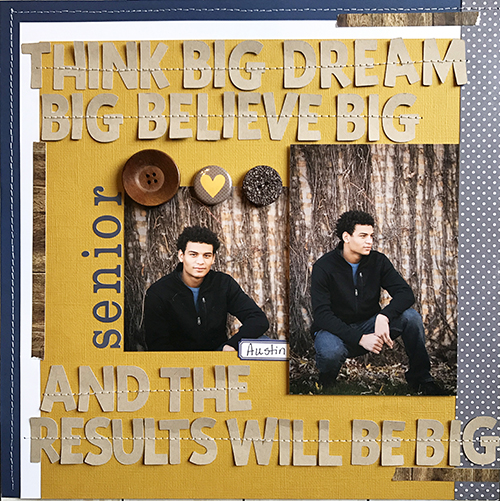This horizontally rectangular poster features a vibrant yellow background with light beige letters that inspire: "THINK BIG DREAM" on the top line, "BIG BELIEVE BIG" on the second, and "AND THE RESULTS WILL BE BIG" across the bottom. It showcases a young man named Austin, who has curly, dark hair. The poster includes two images of Austin: the left image is a full-body shot with him squatting and facing the camera, while in the right image, he's in a similar squatting pose but looking off to his right. He is dressed in a dark black jacket over a light blue shirt and blue jeans. The word "SENIOR" is prominently displayed to the left of these images, along with three button-like icons. The poster has distinct borders, with blue edging featuring white "stitching" on the top, bottom, and left sides, and a gray border with white dots on the right side. This detailed senior portrait creatively emphasizes the motivating text, encapsulating both a personal and aspirational spirit.